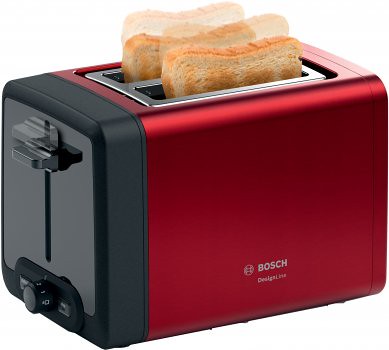This is a detailed product photograph of a contemporary Bosch toaster, set against an all-white background. The toaster itself boasts a modern design with red metallic sides, complemented by dark gray and black trim, and a silver top where the toast pops up. Prominently displayed on the toaster's front in light gray text is the Bosch logo, accompanied by a smaller, unreadable line of text beneath it. The toaster features two slots, currently holding two pieces of golden-brown toast with tan crusts, partially lowered. A unique feature of the image is the ghost-like overlay of the toast above the slots, which creates a sense of motion as if the toast has just been or is about to be ejected. The toaster's left side includes a black paddle for lowering the toast and a black dial at the lower front to adjust the desired level of toasting, likely featuring numerical settings. The photo is slightly angled, allowing a view of both the front and the left side, emphasizing the sleek and functional design of this Bosch toaster.